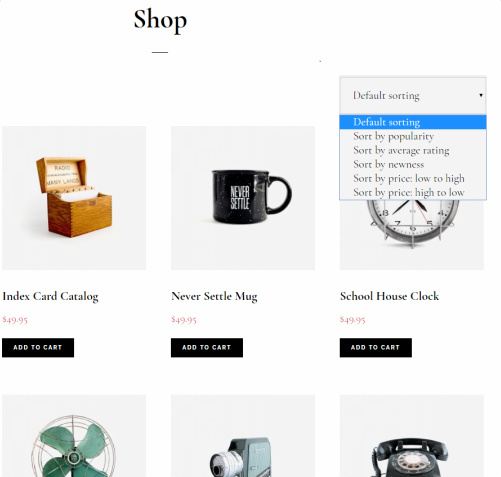The webpage appears to be an e-commerce site with a clean, minimalist design featuring a white background. At the top of the page, the word "Shop" is prominently displayed in black text. The page showcases six items, each with an image, a description, and a price.

1. **Index Card Catalog**: A vintage wooden index card catalog priced at $49.95.
   
2. **Never Settle Mug**: A sleek black coffee mug with the phrase "Never Settle" printed on the side, also priced at $49.95.
  
3. **Schoolhouse Clock**: An antique-style schoolhouse clock available for $49.95.

The bottom three items are partially visible, revealing only the top portions of their pictures and descriptions:
   
4. **Vintage Tabletop Metal Fan**: Showing the top part of an old-time tabletop metal fan.
   
5. **Retro Camera**: The top portion of an old-style camera is visible.
   
6. **Classic Rotary Phone**: The upper part of a vintage tabletop rotary phone is shown.

While the full details and prices of the bottom three items are not visible, it is inferred that they might be priced similarly at $49.95 each.